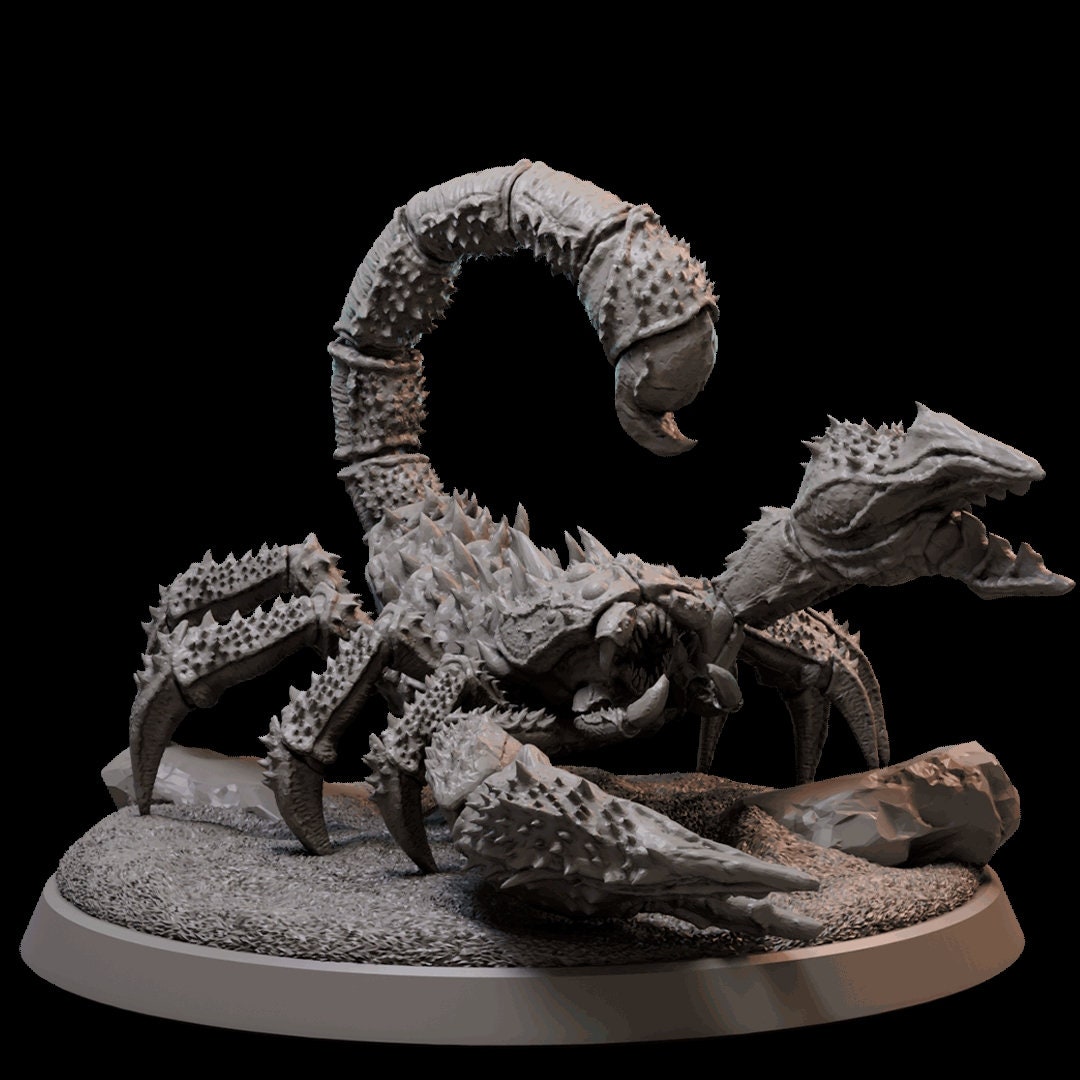This detailed, close-up image showcases a highly detailed scorpion statue set against a stark black background. Crafted from a light gray metal with various shades, the scorpion sits on a circular base of the same material. The base features a textured surface that resembles sand and rocks. 

The scorpion's form is intricately sculpted, with four legs visible on the right side, each adorned with meticulous spikes. The front right claw rests on the ground, while the left claw is elevated, poised for an attack. The scorpion's tail arches up and over its head, ending in a sharply pointed stinger. Its body bristles with additional spikes, more than typically seen on a real scorpion, adding a dramatic flair. 

The statue's geometric precision captures not just the overall form of the scorpion but also minute details like the textures of the legs, the poised, venomous tail, and its prominently featured mouth and pincers. A small rock is discernible on the base's right-hand side, adding to the lifelike environment of this mesmerizing art piece.